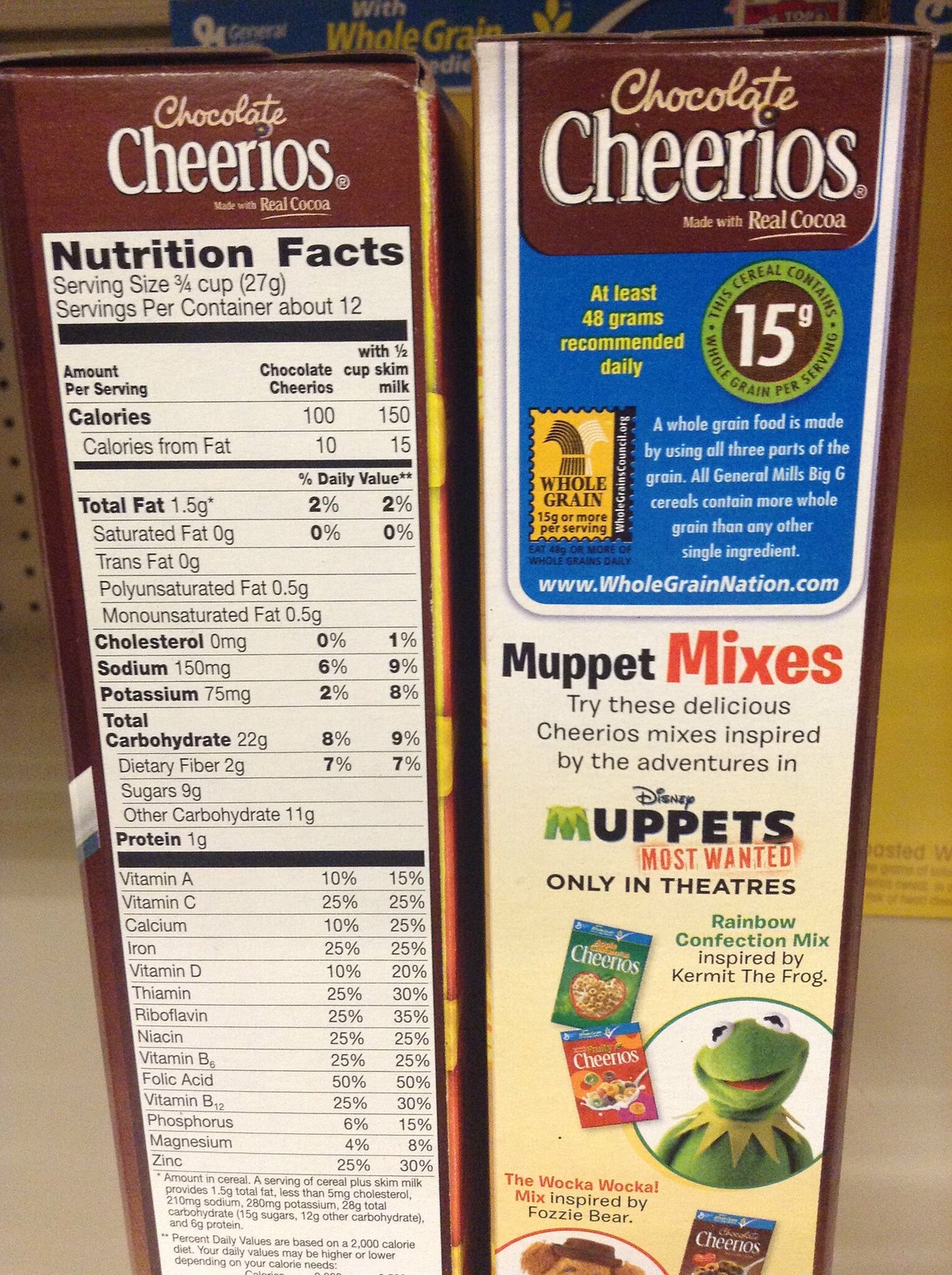The photograph depicts two boxes of Chocolate Cheerios positioned side by side, with each box facing a different direction, thereby revealing both the front and side panels. The box on the left presents the side panel featuring the Nutrition Facts in a black and white format, providing detailed nutritional information. The box on the right displays a side panel brimming with additional information about the cereal, including the number of grams of whole grains per serving. Moreover, this panel introduces other cereals in the "Muppet Mixes" range, inspired by the beloved Muppets characters, and showcases an endearing image of Kermit the Frog.